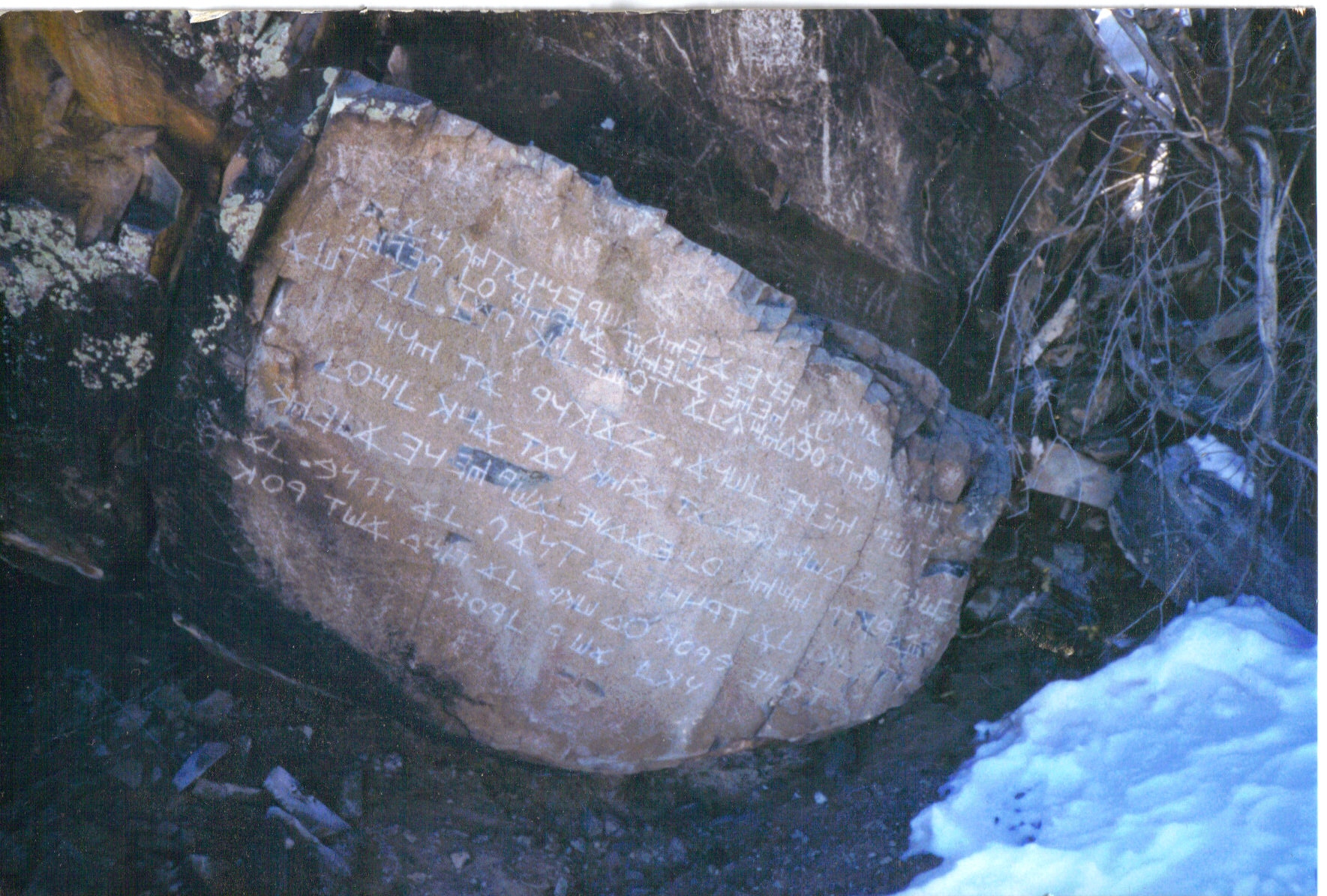This image features an intriguing piece of machinery or a stationary scroll, prominently showcasing a large slab, potentially made of rock or metal. Draping the slab is a brown parchment or covering, adorned with numerous white characters. These characters vary between recognizable letters and numbers and a series of seemingly random shapes, suggesting a complex script or code not in English.

The context of the scene adds depth to the narrative—the background reveals an outdoor setting marked by the natural elements. Visible are the branches of a tree and a dirt floor, indicative of an open, earthy environment. In the bottom right corner, a patch of smooth snow is present, appearing to have been traversed, evidenced by faint footmarks or indentations. Adding to the scene's rustic charm, the upper left portion of the photo captures what looks like a wooden carving, possibly part of the ground setup next to the mysterious device. The overall composition tells a rich story of a possibly ancient or esoteric artifact set against a serene, natural backdrop.